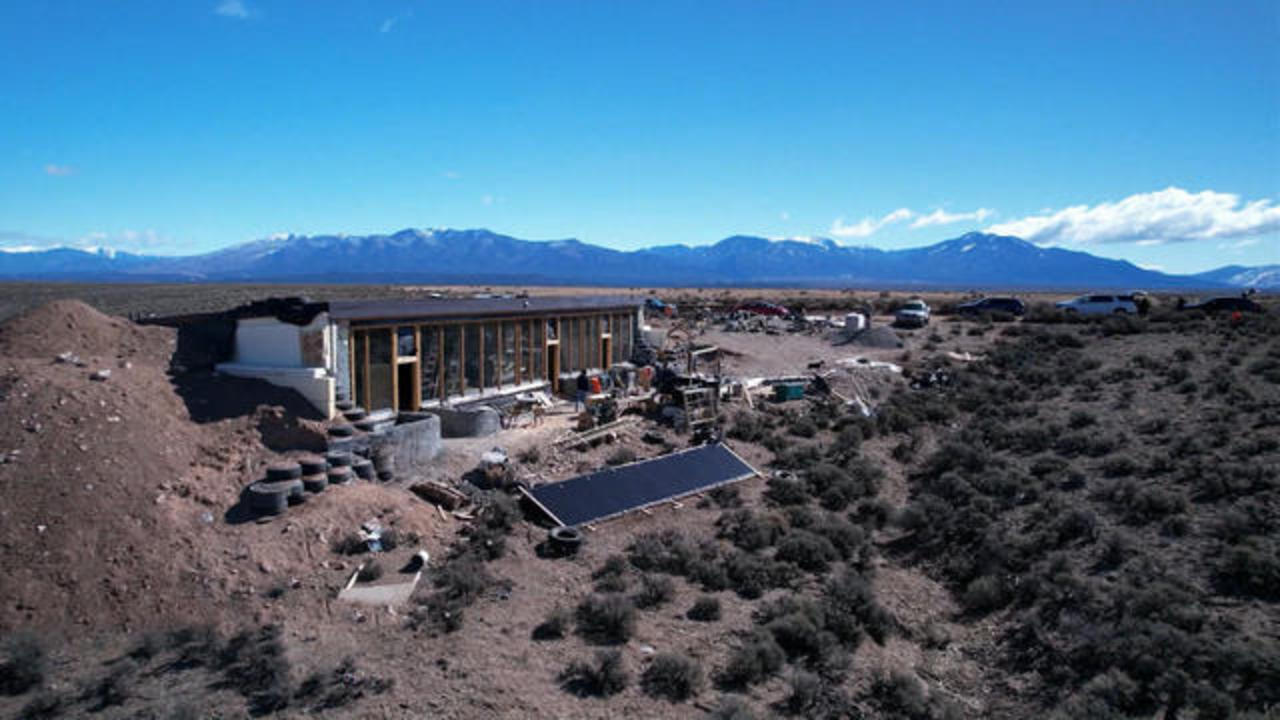This overhead photograph captures an outdoor construction project situated in a desert-like area, framed by a stunning backdrop of a sprawling mountain range under a vivid blue sky with scattered clouds. The focal point of the image is an incomplete building nestled into a hill, which has patches of greenery with bushes and trees dotting the landscape. A prominent solar panel lies on the ground, likely supplying power to the building. Cars are visible nearby, emphasizing the ongoing development. The picture is characterized by a variety of colors including blue, gray, brown, tan, and hints of red, creating a picturesque yet arid setting. The perspective suggests the photo was taken from an elevated position such as a cliff or a taller building, offering a comprehensive view of the site and the diverse natural elements that form its surroundings.